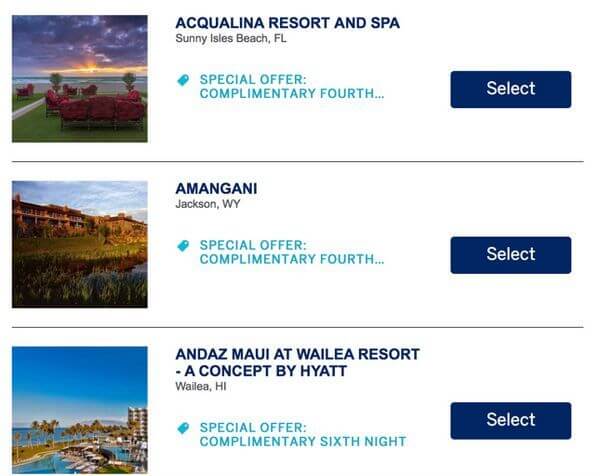The described image webpage boasts multiple distinct sections showcasing luxurious destinations with vibrant visuals and descriptive text. 

On the left-hand side, there's an inviting outdoor seating area featuring a brown couch and red chairs positioned on a lush green lawn, all bordered by a small white wall. This scene is set against a dramatic sky darkened to gray, streaked with captivating purple and orange hues from a setting sun emitting rays of orange and yellow.

On the right-hand side of the page:
1. **Destination One:**
   - **Text**: In bold blue typeface, the words "AQ, ACQ, UA, LINA, Resort and Spa" stand out. Below, in black, the location "Sunny Isles Beach, FL" (Florida) is displayed alongside a cyan blue tag.
   - **Special Offer**: The tag reads "Special Offer: Complimentary fourth night" followed by three ellipses.
   - **Button**: A bold blue rectangular button labeled "Select" in white text.

   Below this text, there's an image of a charming villa, brown in color, amid green grass with its reflection shimmering on the water. Further text states "AM, ANG, ANI" and below it, "Jackson, WY" (Wyoming) in bold blue with the location repeated in black.
   - **Special Offer**: Similar to the first destination, it features a cyan blue tag with "Special Offer: Complimentary fourth night" followed by ellipses.
   - **Button**: A blue "Select" button.

2. **Destination Two:**
   - **Text**: Against the scenic backdrop, bold blue text reads "ANDAZ MAUI AT WAILEA Resort - A concept by HYATT". Beneath that, "WAILEA, HI" (Hawaii) is printed in black.
   - **Special Offer**: The cyan blue tag promises a "Special Offer: Complimentary sixth night".
   - **Button**: A final blue "Select" button.

Each section features evocative imagery and descriptive text, offering visual and textual allure to potential visitors.